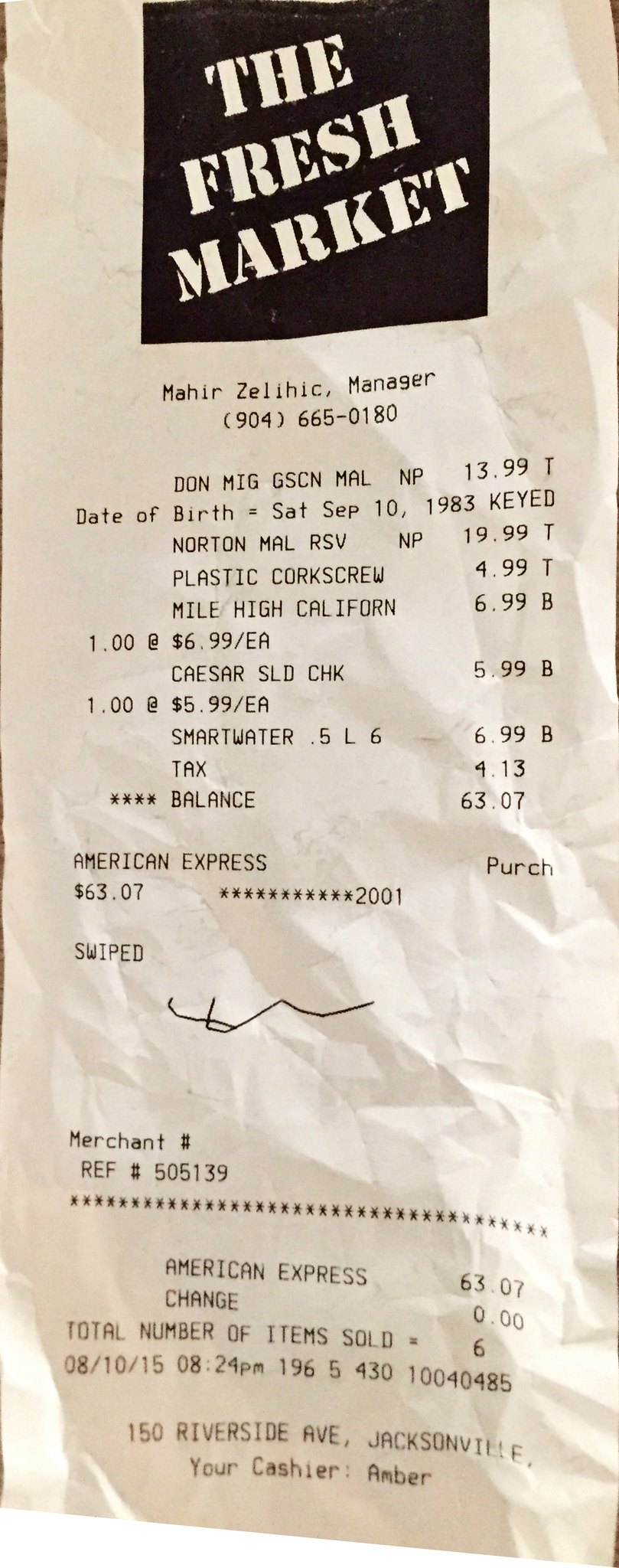A detailed photograph of a wrinkled receipt from the Fresh Market. The receipt is oriented vertically, with the Fresh Market logo prominently displayed at the top center. Directly below, it lists "Menhir Zellheit, Manager" along with a contact phone number: 904-665-0180. The list of purchased items includes a plastic corkscrew, Mile High California, Caesar’s Salad, and Smart Water. The total purchase price is $63.07, paid using an American Express card. The receipt shows a merchant reference number of 505-139 and notes that the transaction was processed at 8:24 PM on 08/10/15. It also indicates that a total of six items were sold. At the bottom, the receipt provides the store's address: 150 Riverside Ave, Jacksonville, FL, and names Amber as the cashier. The receipt confirms that no change was given, as the total amount due was fully covered by the payment.